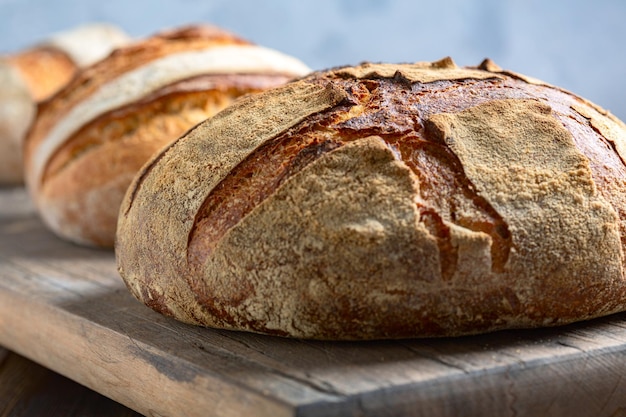This rectangular photograph, approximately four to five inches wide and three inches high, captures three round, freshly baked loaves of bread on a rustic wooden table. The table, which appears dusty and has beveled edges, angles from the center left toward the lower right-hand side of the image.

The loaf in the foreground is the most prominent, featuring a dark, crusty top with a light dusting of flour and deep crosshatches, creating an appealing rugged texture. The crack on its surface reveals a more appetizing, natural brown interior. 

Behind it, a second loaf, with a reddish-brown crust, sports a single, prominent crack that runs from one end to the other. This loaf is slightly lighter in color than the front one and is also clearly visible.

At the back, there is a third, less distinct loaf that appears blurry, with only hints of white and brown visible. The loaves sit very close together, maximizing the use of the limited space on the table.

The background features a blurred gradient of grayish-blue hues, drawing attention to the bread while suggesting a cool environment, possibly indicating that the loaves are being cooled.